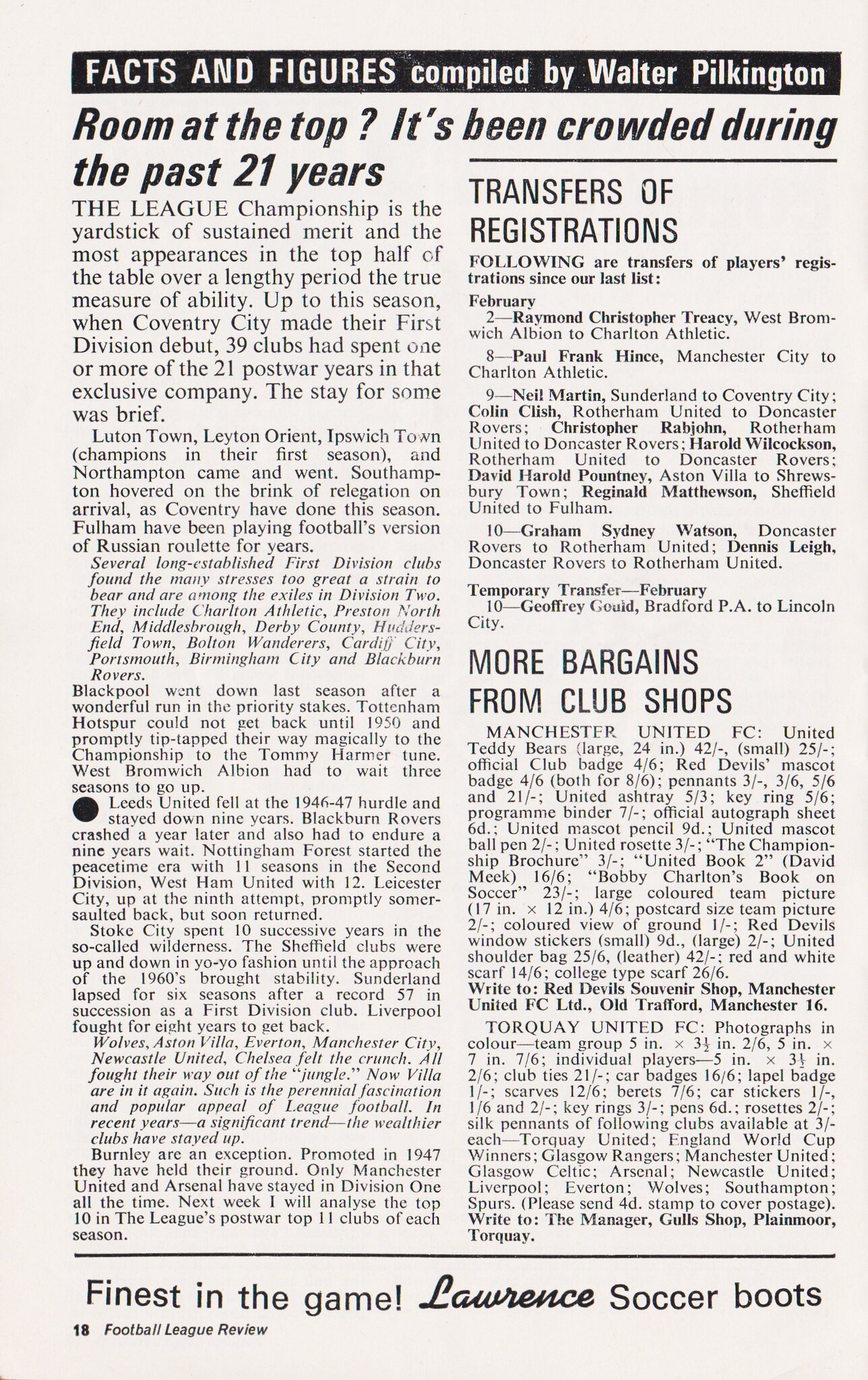This black-and-white page from "Football League Review," marked as page 18 in the bottom left corner, is a detailed section rich with football information. At the very top, a black horizontal bar with white all-capital letters announces "Facts and Figures," compiled by Walter Pilkington. The main article, titled "Room at the Top?" in bold, examines the league championship over the past 21 years, highlighting the consistent performers among the 39 clubs that have spent time in the top-flight since the post-war period. This comprehensive analysis comprises numerous paragraphs arranged in a two-column format. On the right-hand side, two additional sections provide further insights: "Transfers of Registrations," listing player movements between clubs, and "More Bargains from Club Shops," detailing items for sale at various football club stores. At the very bottom, a single line of text advertises "Finest in the Game! Lawrence Soccer Boots," with "Lawrence" emphasized in bold italic font. The overall layout and typographic choices indicate a traditional print publication style.